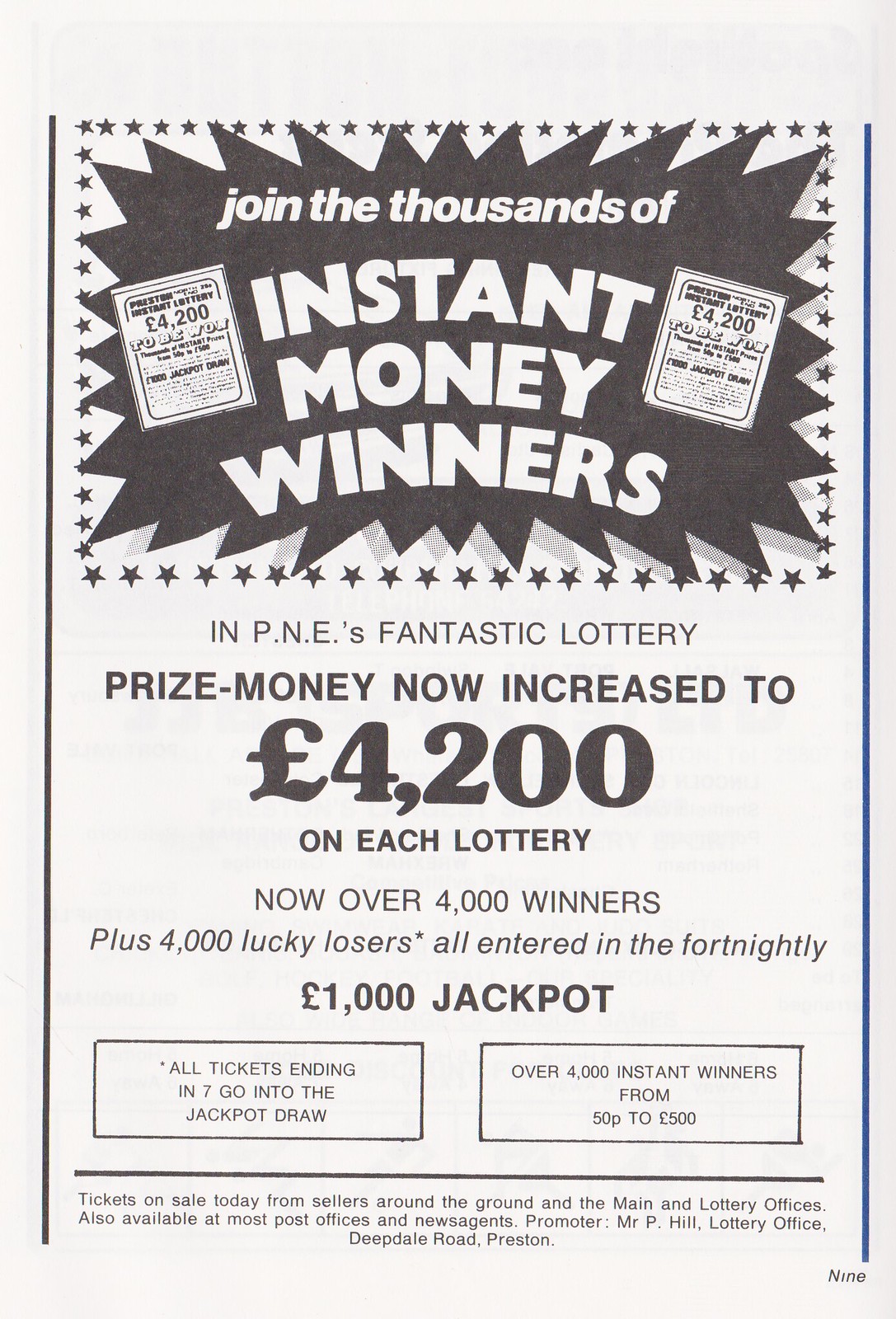The image is an old black and white advertisement poster with text predominantly set against a light-green background. At the top of the poster, a large black star frames the white text, "Join the thousands of instant money winners." This main message is surrounded by smaller black stars and flanked by lottery tickets on each side. Below it, detailed text describes P&E's Fantastic Lottery, announcing that the prize money has now increased to £4,200 per lottery. It highlights that there are over 4,000 winners, plus an additional 4,000 "lucky losers" who are entered into a fortnightly £1,000 jackpot. Notably, all tickets ending in 7 are automatically entered into this jackpot draw. The ad further mentions that there are over 4,000 instant winners, with prizes ranging from 50 pence to 500 pounds. It specifies that tickets are on sale from sellers around the ground, the main and lottery offices, and are also available at most post offices and newsagents. The promoter of the lottery is Mr. P Hill, with the Lottery Office located on Deepdale Road, Preston, issue 9. The design of the poster is straightforward and text-heavy, with lottery cards visually supporting the text at the top.